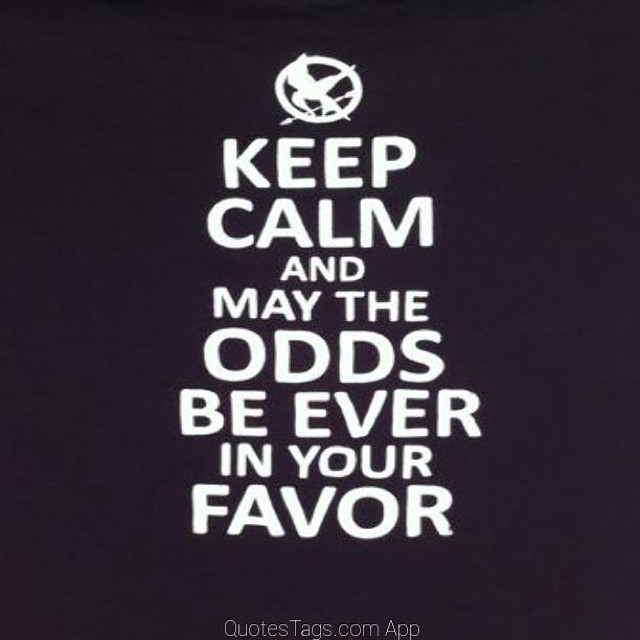The image features a square, predominantly black background, possibly dark gray, with large white text in the center that reads, "KEEP CALM AND MAY THE ODDS BE EVER IN YOUR FAVOR," playing on the "Keep Calm and Carry On" slogan. The text varies in size: "KEEP CALM" and "ODDS" are in a larger font, while "AND," "MAY THE," and "IN YOUR" are smaller. At the top, there's a white circle containing a bird with wings spread, reminiscent of the Hunger Games Mockingjay pin, complete with an arrow. At the bottom, it says "QuotesTags.com app," with "Quotes" and "Tags" both capitalized. The font used has soft edges but is very plain and bold.